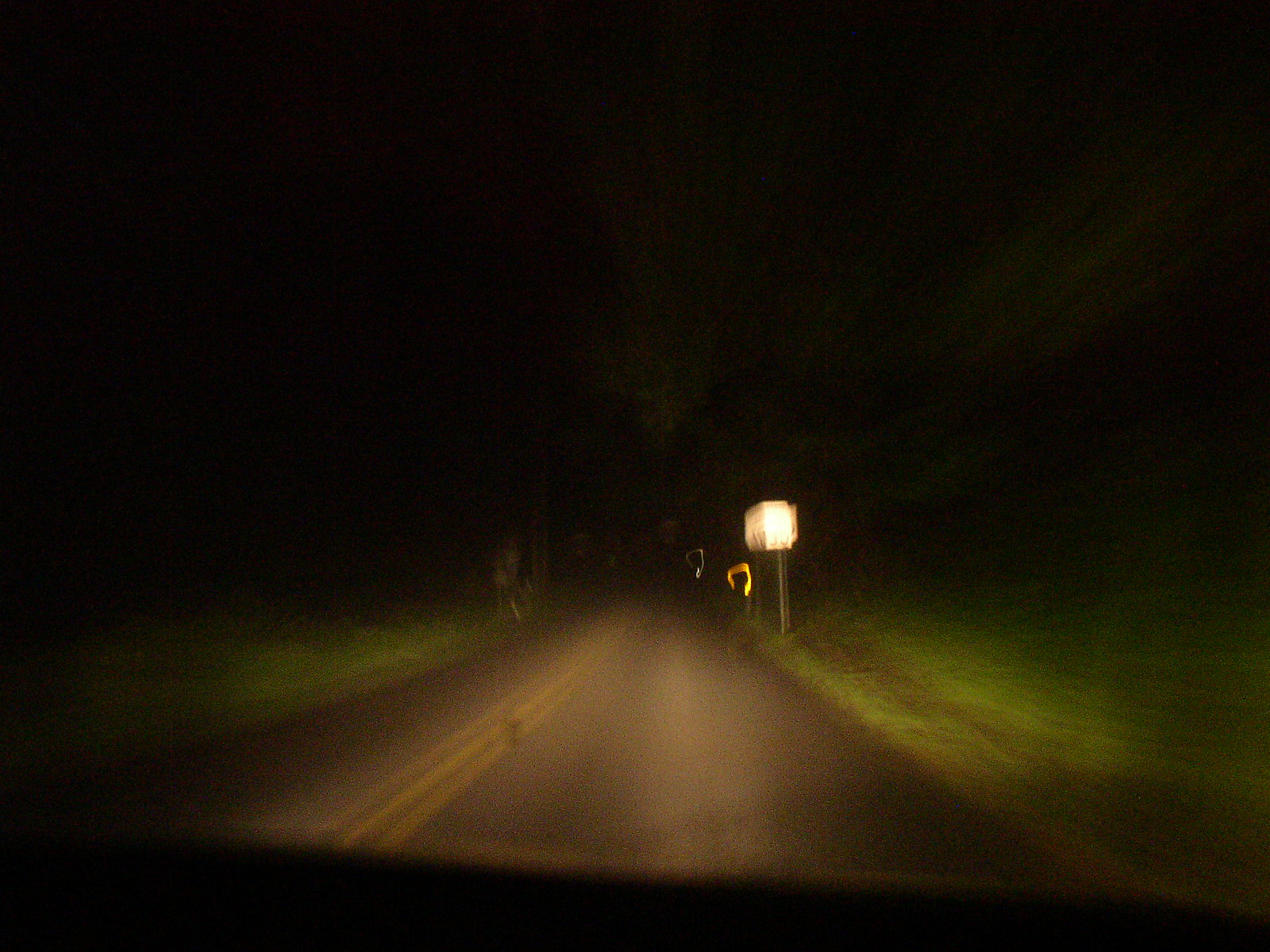In this rectangular photograph, taken on a dark, murky night, we are peering through the windshield of a vehicle, evidenced by the black dashboard visible at the bottom of the image. The scene is a rural, one-lane each-way road, dimly illuminated by the car's headlights. A trio of slender yellow stripes marks the center of the road, dividing the two-way traffic. On the right side of the road, a white sign stands on a post, although it is blurred and difficult to discern. Across from it, on the left, there appears to be either a mailbox or some small structure halfway up the image, though its exact nature is unclear due to the poor focus. The right side of the road reveals a patch of grass brightly lit by the headlights, contrasting with a narrower, dimly lit strip of grass running along the left side.